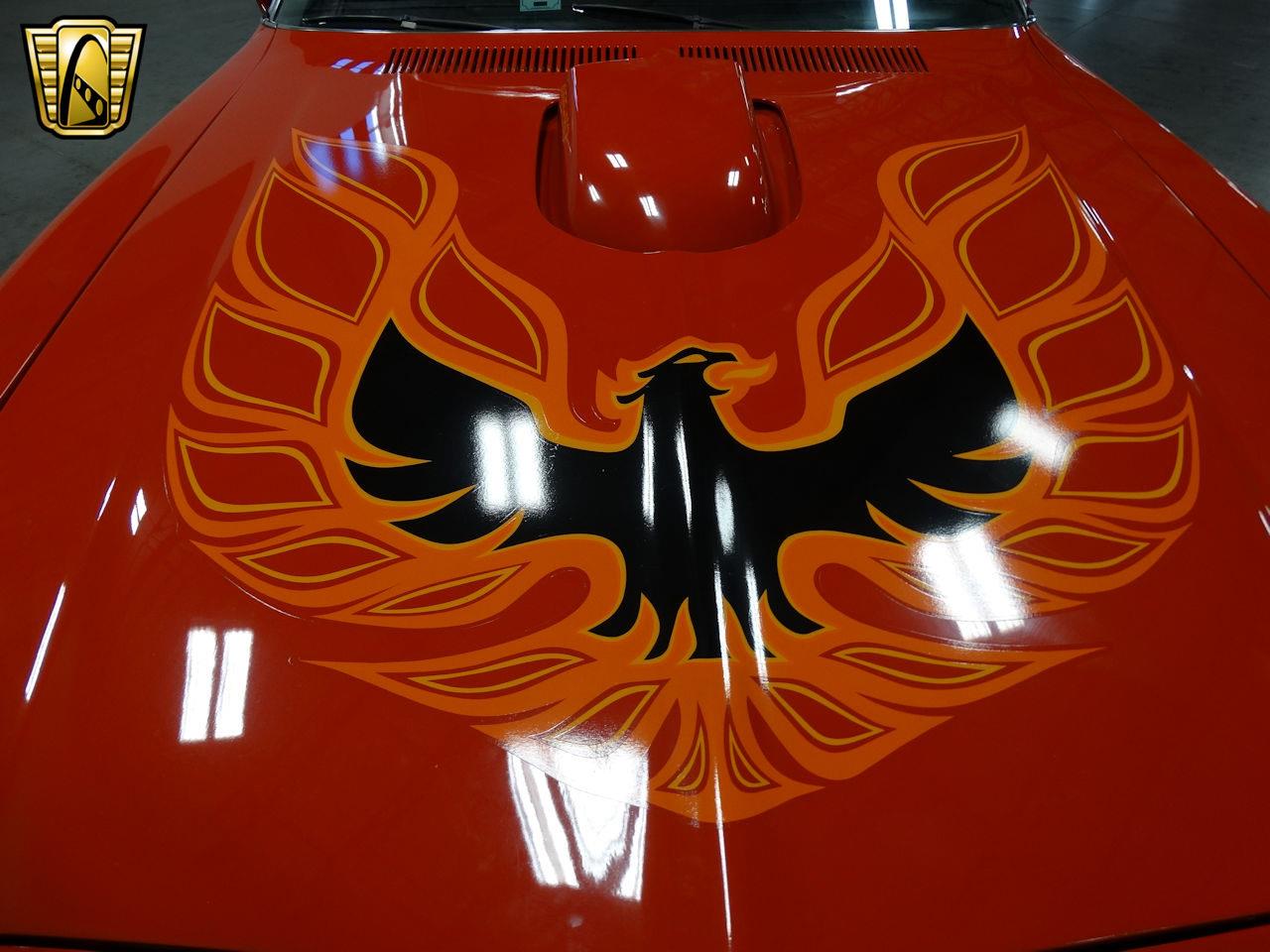The image is a close-up photograph of the shiny, dark maroon hood of a muscle car, almost certainly a Firebird, given the prominent emblem. This emblem features a dynamic design of a black bird with wings that resemble flames, rendered in orange and yellow hues. The bird, possibly a phoenix, is depicted open-mouthed and seeming to breathe fire. The hood, which takes up nearly the entire frame, reflects a lot of light, likely from long fluorescent bulbs above, lending to its extremely glossy appearance. Near the upper left-hand corner of the photo, there's an additional emblem that looks like a stylized golden steering wheel inside a rectangular box. This high-resolution image is well-centered and clear, suggesting a setting such as a garage, dealership, or car meet, where enthusiasts might admire such vehicles. Overall, the photograph captures the intricate details and vibrant colors of the Firebird emblem against the immaculate, polished surface of the car's hood.